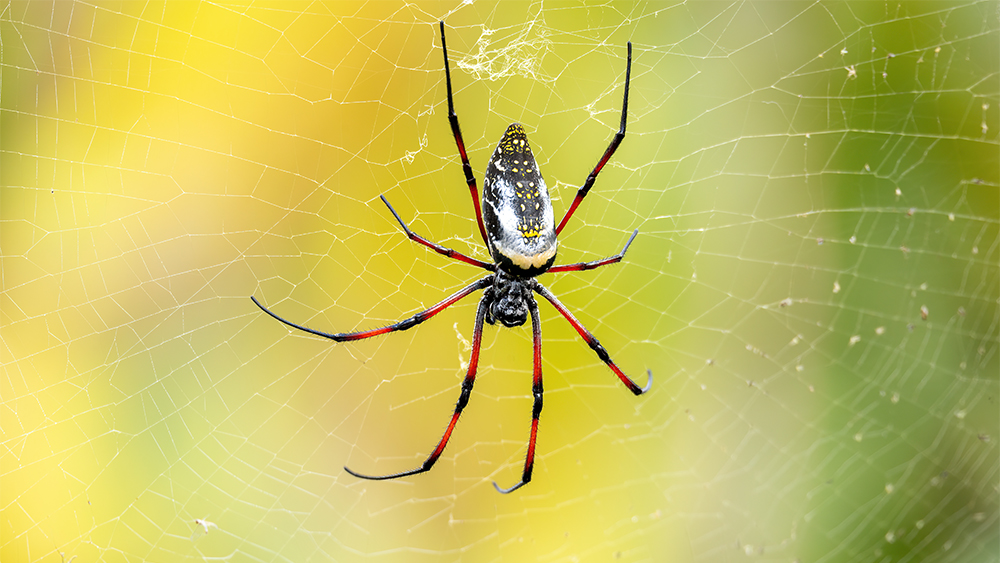This detailed photograph captures a spider clinging to its intricate web, facing downward with its body prominently displayed in the center of the image. The spider, with its eight long legs segmented with alternating red and black joints, features a striking black head and an oval-shaped abdomen that tapers towards the back. Its back showcases a vivid pattern comprising white, gray, and yellow spots as well as rows of dots that resemble eyes, though they are merely body markings. The webbing spans the entirety of the frame, illustrating intricate patterns from edge to edge. The background is blurred into a wash of greens and yellows, with a distinct green border on the right, suggesting an outdoor setting. This close-up emphasizes the spider's detailed coloration and the elaborate structure of its web against a softly colored backdrop.